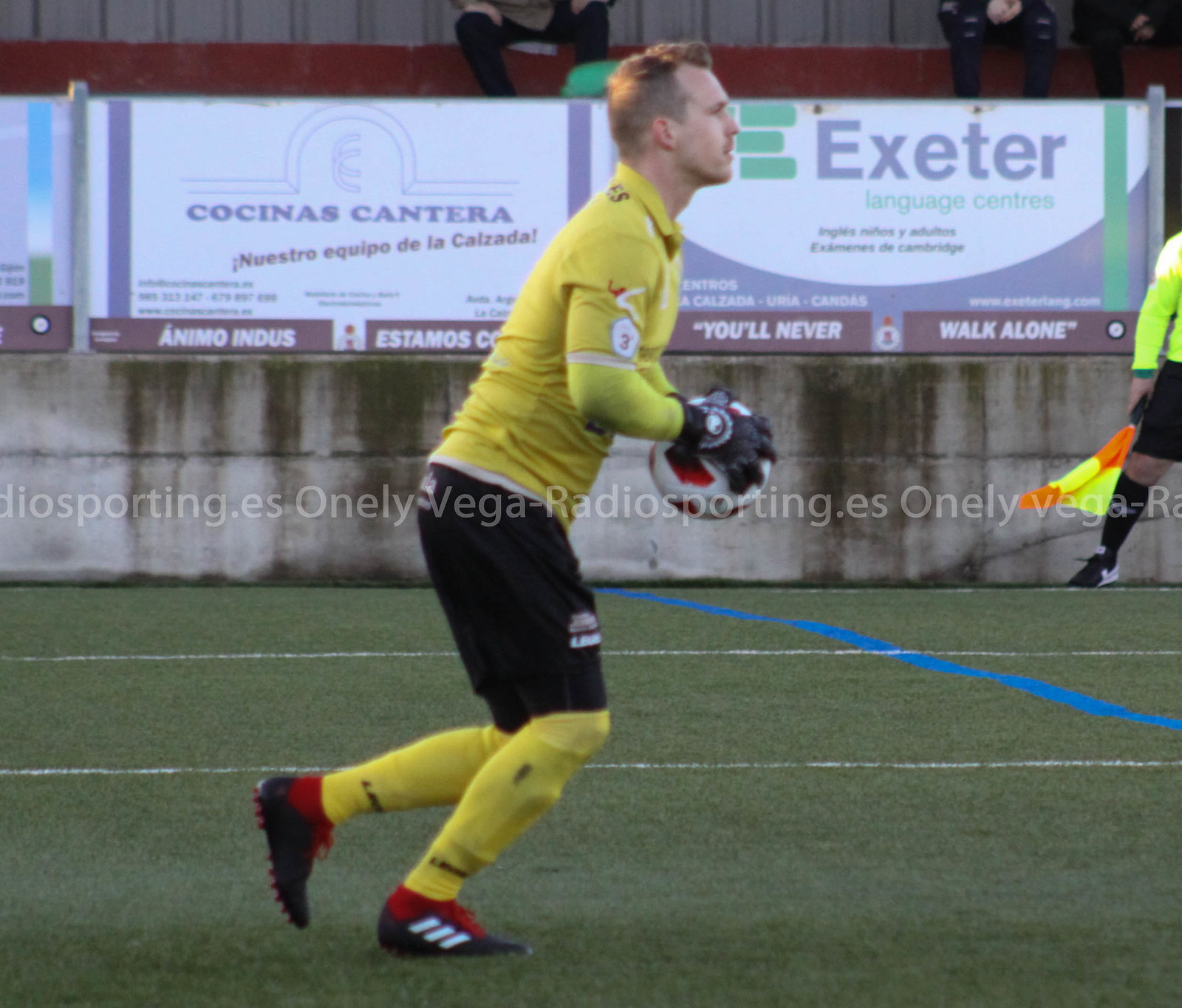This image captures a close-up action shot of a soccer goalie (European football goalkeeper) in bright, vivid detail. The goalie, identifiable by his yellow jersey with the number three on it, black shorts, and yellow socks pulled over shin guards, is dynamically caught in motion. He is sprinting towards the right side of the frame, gripping the soccer ball firmly with both gloved hands at his stomach, ready to make a play. His footwear includes distinctive black and white Adidas cleats, featuring three white stripes.

The background shows a grass field marked with various white lines, including horizontal and a solitary vertical blue line intersecting them. Behind the field, the stands are populated with a few spectators and adorned with several signs, including a prominent "Cosinus Cantera" and "Exeter Language Centers." The lower portion of the backdrop consists of a weathered light and dark brown streaked stone wall. Near the right edge of the image, part of another figure – likely a match official or linesman – is visible. This person is dressed in a long-sleeved yellow shirt and holds an orange and yellow flag, contributing to the rich, dynamic tableau of this sporting moment.